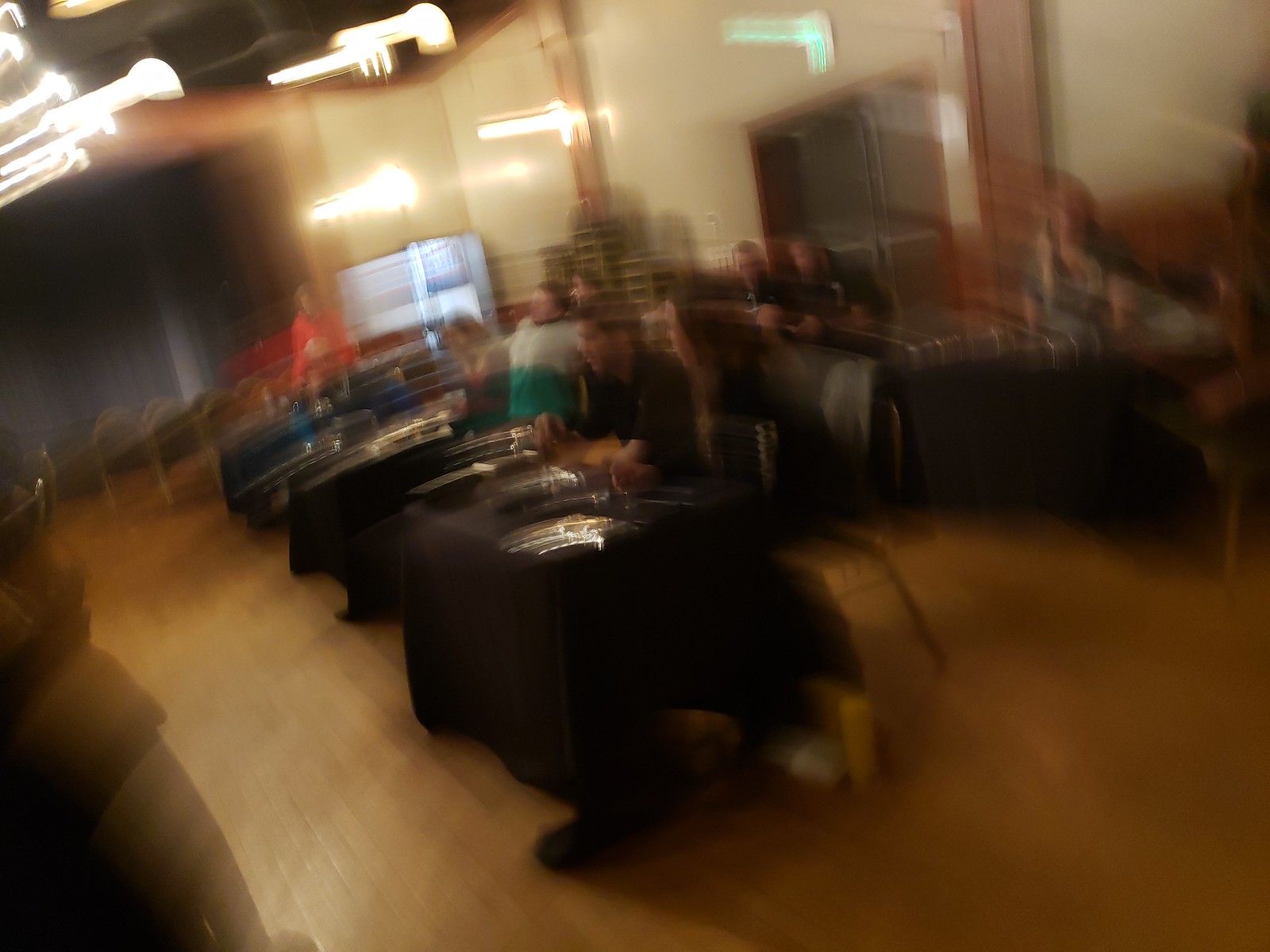In this photograph, a blurry image captures a large room that could either be a conference hall, a casino, or a meet-and-greet event. Several small tables, each draped with black tablecloths, are arranged across a light-colored wooden floor. People are seated on one side of the tables, seemingly waiting to engage in conversations, suggesting that this could be a job recruitment event or a similar setup. Though the details are difficult to discern due to the blurriness of the photo, the general layout and activity suggest a formal, organized gathering. No text accompanies the image.